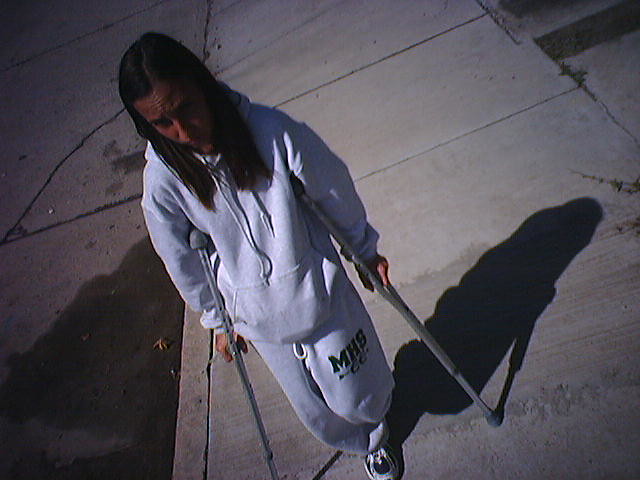In this grainy, security camera-like photograph, a mid-teen girl with long, dark brown hair parted down the middle is depicted. She is wearing a light gray hooded sweatshirt with long drawstrings and matching light gray sweatpants featuring the letters "MHS" in green block letters, along with "CC" and an arrow indicating a high school cross-country team. The girl's face shows a furrowed brow, expressing unhappiness as she looks straight ahead, not at the camera. She is utilizing silver crutches with gray rubber traction tips and cushioned arm supports, holding her left leg up behind her, suggesting an injury, likely from running. Her footwear consists of white shoes with some black fabric near the toes. She casts a shadow to her right on a light gray sidewalk and stands near the edge of a similarly light gray road. The angled photo shows her feet at the bottom with the landscape tilting about 30 degrees to the left, including a visible street puddle. The scene is dimly lit, despite being taken during the day.